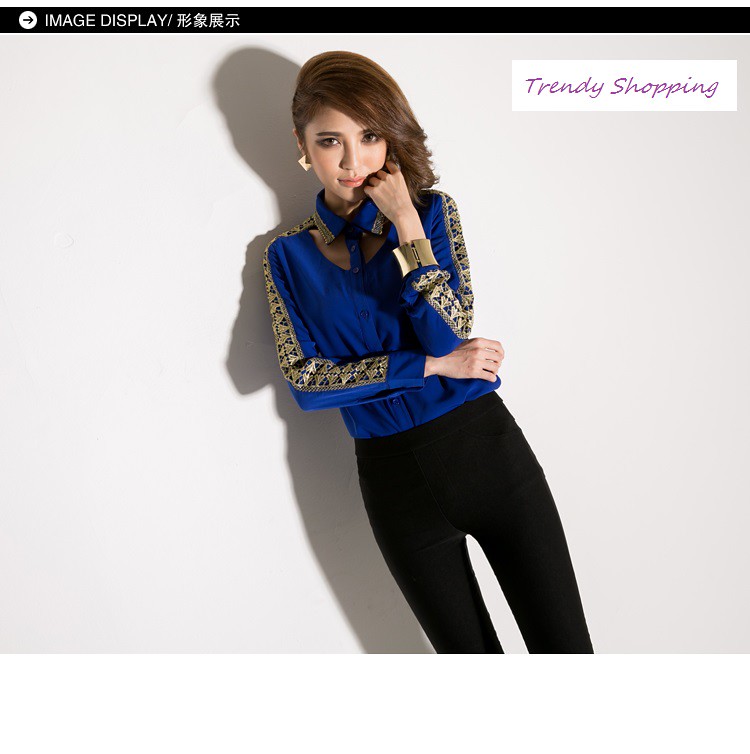The photograph showcases a female model, likely in her 20s or 30s, standing against a white background. She has dark brown hair styled to cover her left ear while her right ear, adorned with an earring, is visible. Her hair is swept to the left, and she gazes directly into the camera with her left hand positioned near her face. The model is dressed in a form-fitting outfit: a blue long-sleeve shirt with gold trim on the shoulders and neck, paired with black pants. Her poised stance casts a shadow on the white background, adding to the image's clean composition. At the top of the image, a black bar runs across the screen, displaying the text "image display" alongside some Chinese characters. Positioned in the top right corner, "trendy shopping" is written in purple cursive within a white box. The model's makeup is subtly applied, enhancing her features and adding to the overall polished aesthetic of the photograph.